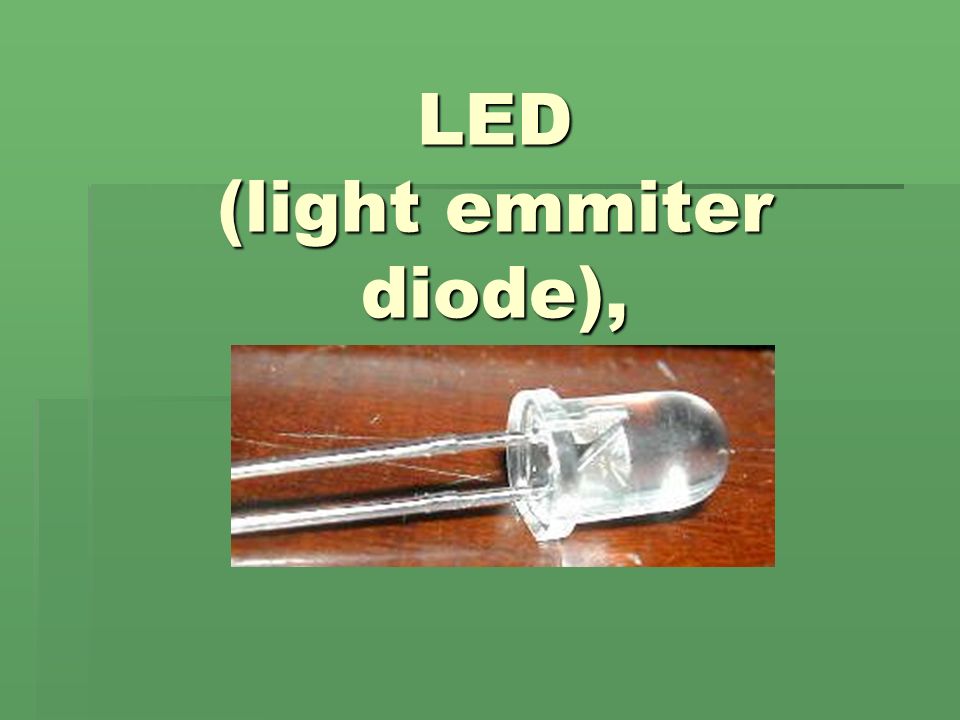The image features a small, classic LED (Light Emitting Diode) positioned at the center of a horizontal rectangular section. This section is embedded within a larger square image that has a prominent green background. The LED itself, clear and whitish in color, has two thin wires extending from its base, ready to be connected to a circuit board. The diode is placed on a scratched, dark brown wooden tabletop, where the wood grain and texture are clearly visible. At the top of the green background, aligned in the center, are the large, light green capital letters "LED" followed by the parentheses containing the words "light emitter diode," explaining the object in the image.